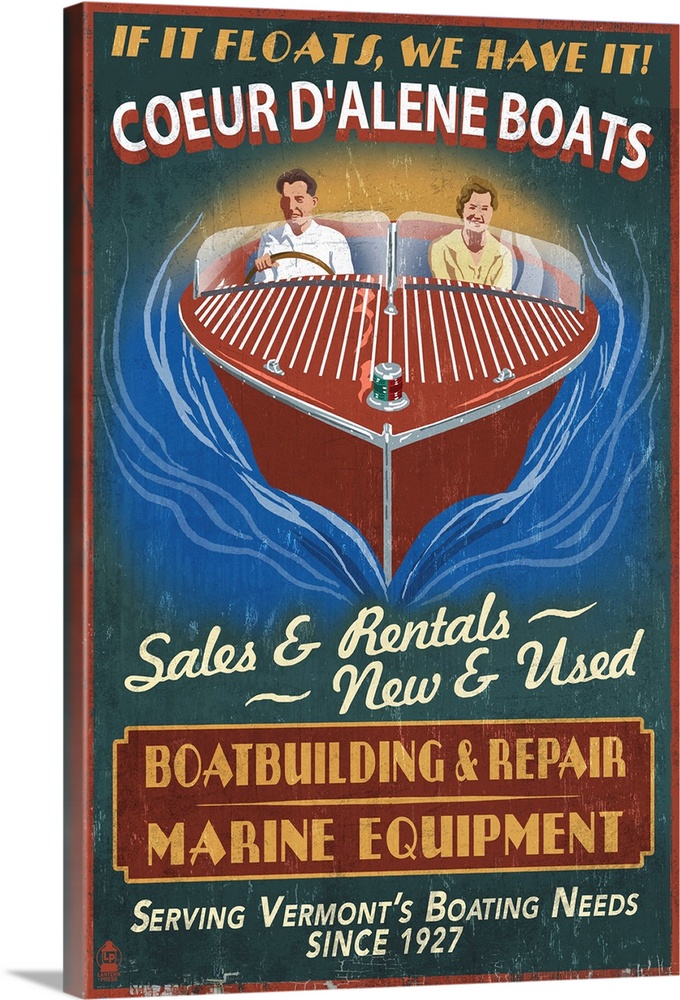The image is a vibrant vintage-style advertisement poster set against a dark green background, resembling a painted metal sign with no border. At the very top, a bold yellow font announces, "If it floats, we have it," followed by slightly arced white and red-shadowed text proclaiming "Kurdaleen Boats." Below this, a retro illustration features a man in a white button-down shirt steering a small, red boat with silver trim and vertical white lines. A woman beside him, in a yellow top with short brown hair, exudes joy as they glide through the water. The scenic background includes waves and a hint of the sun on the horizon. The lower part of the image contains cream-colored text stating, "Sales and rentals, new and used." Below this, a red banner with gold outlining reads, "Boat building and repair, marine equipment." Finally, the poster concludes with the phrase, "Serving Vermont's boating needs since 1927."